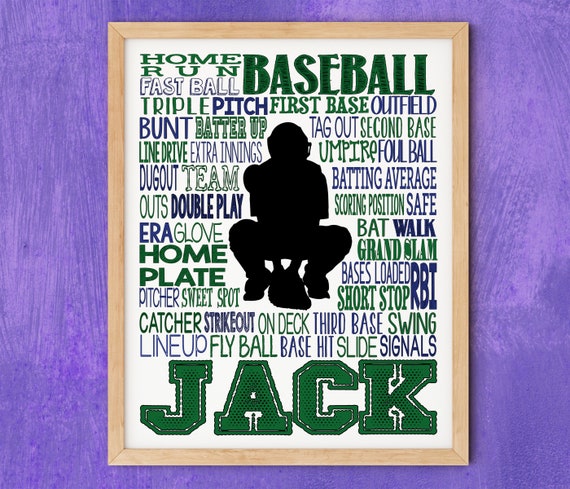Set against a light purple background with visible brush strokes, this slightly rectangular poster, approximately four inches wide and three inches high, is framed in a thin light beige wood. The poster itself features a central figure, a black silhouette of a baseball catcher squatting down with a catcher's mitt held between their feet, and a mask clearly visible on their head. Surrounding the silhouette, in a vibrant mix of green and blue lettering, are numerous baseball-related terms forming a dense collage. Key phrases include "home run," "fastball," "baseball," "triple pitch," "first base," "outfield," "bunt," "batter up," "tag out," "second base," "line drive," "extra innings," "umpire," "foul ball," "dugout," "team," "batting average," "outs," "double play," "scoring position," "safe," "ERA," "glove," "bat," "walk," "home," "grand slam," "plate," "bases loaded," "pitcher," "sweet spot," "shortstop," "RBI," "catcher," "strikeout," "on deck," "third base," "swing," "lineup," "fly ball," "base hit," "slide," and "signals." Dominating the bottom of the poster in large green letters is the name "JACK."